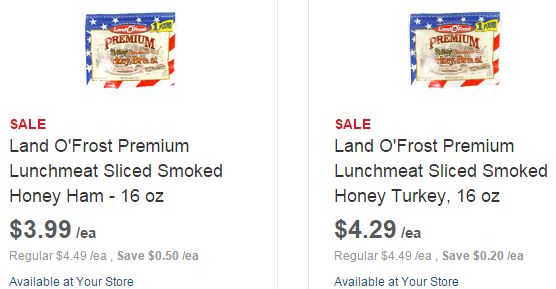This image features two side-by-side sale advertisements for Land O'Frost Premium Lunch Meat from a store. Each advertisement showcases a small thumbnail of the product above detailed descriptions of the sale items.

- **Left Advertisement**: 
  - **Product**: Land O'Frost Premium Sliced Smoked Honey Ham 
  - **Weight**: 16 ounces 
  - **Sale Price**: $3.99 each 
  - **Regular Price**: $4.49 each 
  - **Savings**: Save 50 cents each 
  - **Availability**: Available at your store 
  - **Design**: The text is displayed on a plain white background in black letters, with the word "sale" prominently highlighted in red.

- **Right Advertisement**:
  - **Product**: Land O'Frost Premium Sliced Smoked Honey Ham
  - **Weight**: 16 ounces
  - **Sale Price**: $4.29 each
  - **Regular Price**: $4.49 each
  - **Savings**: Save 20 cents each
  - **Availability**: Also available at your store
  - **Design**: Similar to the left advertisement, the text is on a plain white background in black letters, with the word "sale" in red.

Both advertisements are designed similarly, providing clear, concise information about the discounted prices and the savings customers can expect.